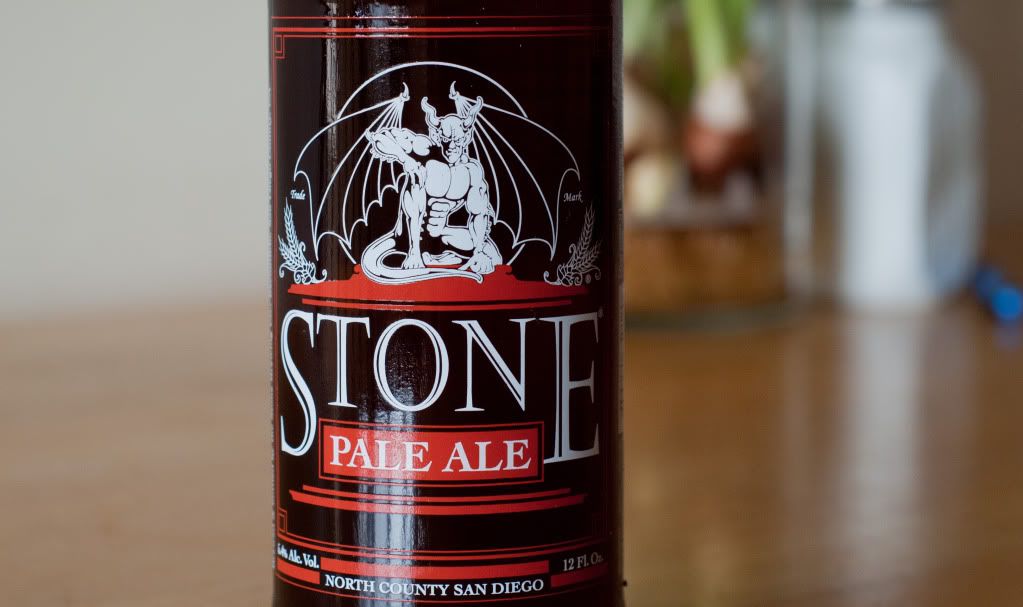The image showcases the bottom half of a beer bottle from Stone Brewery, predominantly featuring its intricate design and label details. The focus is sharply on the bottle, with a blurred wooden table and indistinct background. The bottle has a prominent red and white color scheme with a brown glass body. The central design includes a striking illustration of a gargoyle or demonic figure, depicted in white against a mainly black backdrop with detailed black wings. Below the gargoyle, the word "STONE" is prominently displayed in white. A red rectangle with "PALE ALE" written in white text is situated beneath it. Further down, the label reads "North County, San Diego," with specifics such as alcohol volume and "12 fluid ounces" noted in white text alongside red accents. There is also a watermark from Photo Bucket overlaying the image, stating "Protect more of your memories for less!"